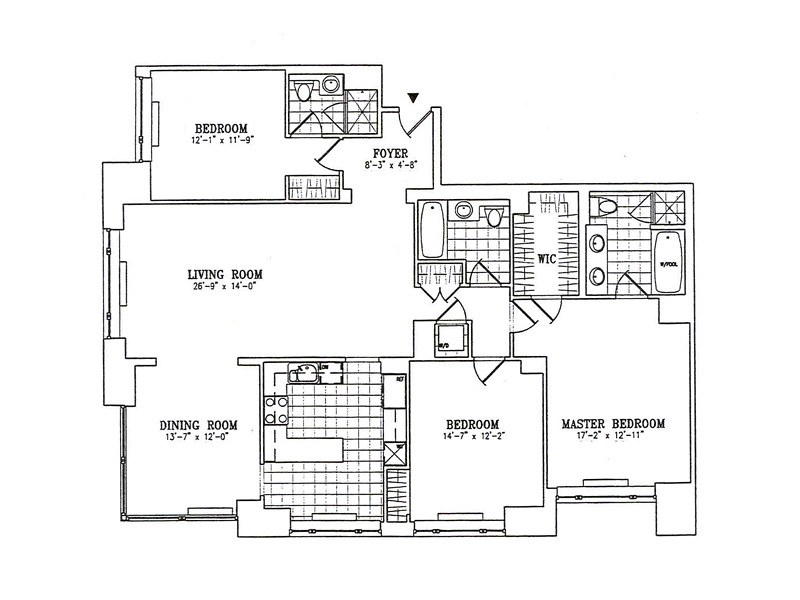This image depicts a comprehensive aerial view blueprint of a room design, typically used for construction or spatial planning purposes. The aspect ratio of the blueprint is slightly wider than it is tall, set against a completely white background, making the edges indistinguishable.

At the center of the blueprint, we observe a detailed layout of various rooms, each drawn with approximate dimensions, albeit some values are difficult to discern. Starting from the upper left corner, we see a square-shaped bedroom, though its exact dimensions are unclear. To the right of the bedroom, there's a smaller and narrower foyer, completing the upper left-hand rectangle of the plan.

Occupying the rest of the space below this rectangle, a large living room is situated in the upper left quadrant of the larger lower section. Meanwhile, the upper right quadrant features several rooms, though not all are labeled. Among these, there are two bathrooms with a room labeled "wick" positioned between them. Additionally, there's an area resembling a hallway.

The lower left quadrant of the layout includes the dining room. Immediately to the right of the dining room, there's an unlabeled room. The right half of the lower section is dominated by the master bedroom, which also slightly extends into the lower right part of the upper right quadrant.

Each room is meticulously plotted to give a rough estimate of their size and spatial relationship to one another, providing an essential guide for construction or planning activities.